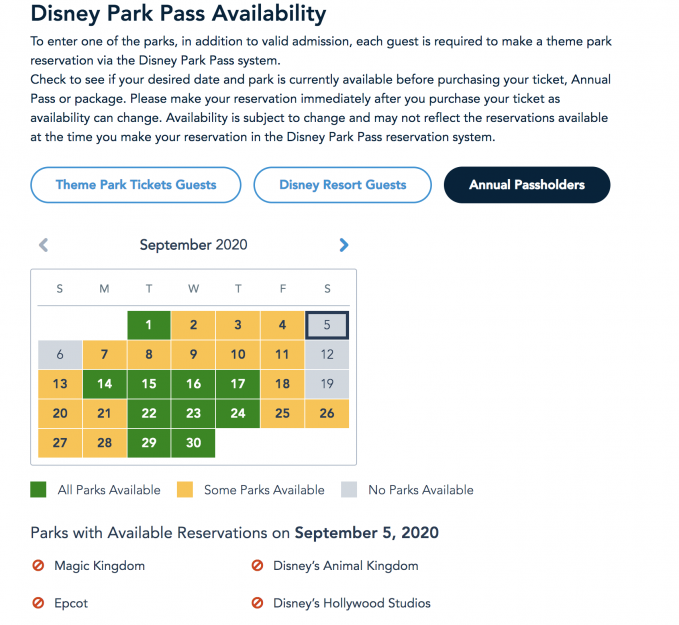The image is a cropped screenshot, either from a tablet or desktop, displaying a page dedicated to Disney Park Pass availability without the visibility of the browser or operating system. The text presented on the page is primarily in black, conveying essential details regarding the process for securing theme park reservations. It states that, in addition to valid admission, each guest must make a theme park reservation through the Disney Park Pass system. Guests are advised to check the availability of their desired date and park before purchasing their tickets, annual passes, or packages. Upon purchasing their tickets, guests must immediately make reservations as availability can change frequently and may not reflect the real-time reservations at the moment of booking in the system.

The page categorizes guests into three types: Theme Park Ticket Guests, Disney Resort Guests, and Annual Pass Holders. At the bottom of the screenshot, a calendar for September 2020 is visible, color-coded to indicate the reservation status: green for all parks available, yellow for some parks available, and gray for no parks available.

For September 2020, the date highlighted is September 5th, showing that no parks have availability on that day. The dates with no availability (gray) are the 5th, 6th, 12th, and 19th. The dates with some parks available (yellow) are the 2nd to the 4th, 7th to the 11th, 13th, 18th, 20th, 21st, and 25th to the 28th. Dates with all parks available (green) are the 1st, 14th to 17th, 22nd to 24th, and the 29th and 30th.

This detailed depiction aids users in determining the best date to make their reservations to visit the Disney Parks.